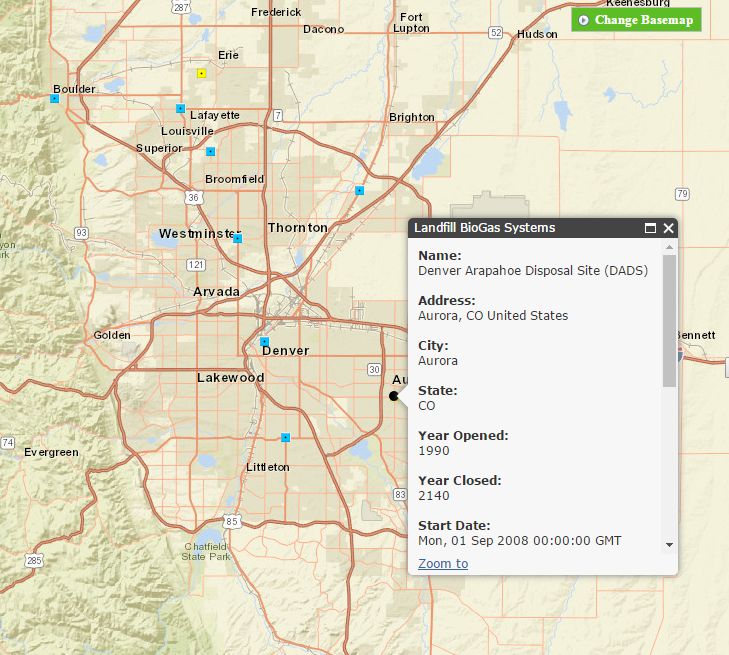This image is a screenshot from a mapping application. The primary view shows a detailed map of the Denver, Colorado area, with various town and city names labeled, including Erie, Lafayette, Louisville, Superior, Boulder, Broomfield, Thornton, Brighton, Fort Lupton, Hudson, Denver, Lakewood, Littleton, Evergreen, Arvada, Golden, Westminster, Frederick, Dacono, and Keenesburg at the very top. 

A prominent black-and-white information box overlays the map, displaying specific details about a facility named "Denver Arafo Disposal Site". It is identified as a landfill biogas system. Additional details include:
- Address: Aurora, CO, United States
- City: Aurora
- State: CO
- Year Opened: 1990
- Year Closed: 2140
- Start Date: Monday, 01 September 2008 at 00:00 GMT

The box also contains a clickable link labeled "Zoom To."

At the very top of the screen, there is a green banner with the text "Change Base Map," offering an option for users to switch the map view. The map background reveals an array of interlinked towns and cities in the vicinity, presenting a comprehensive spatial context for the location data provided.